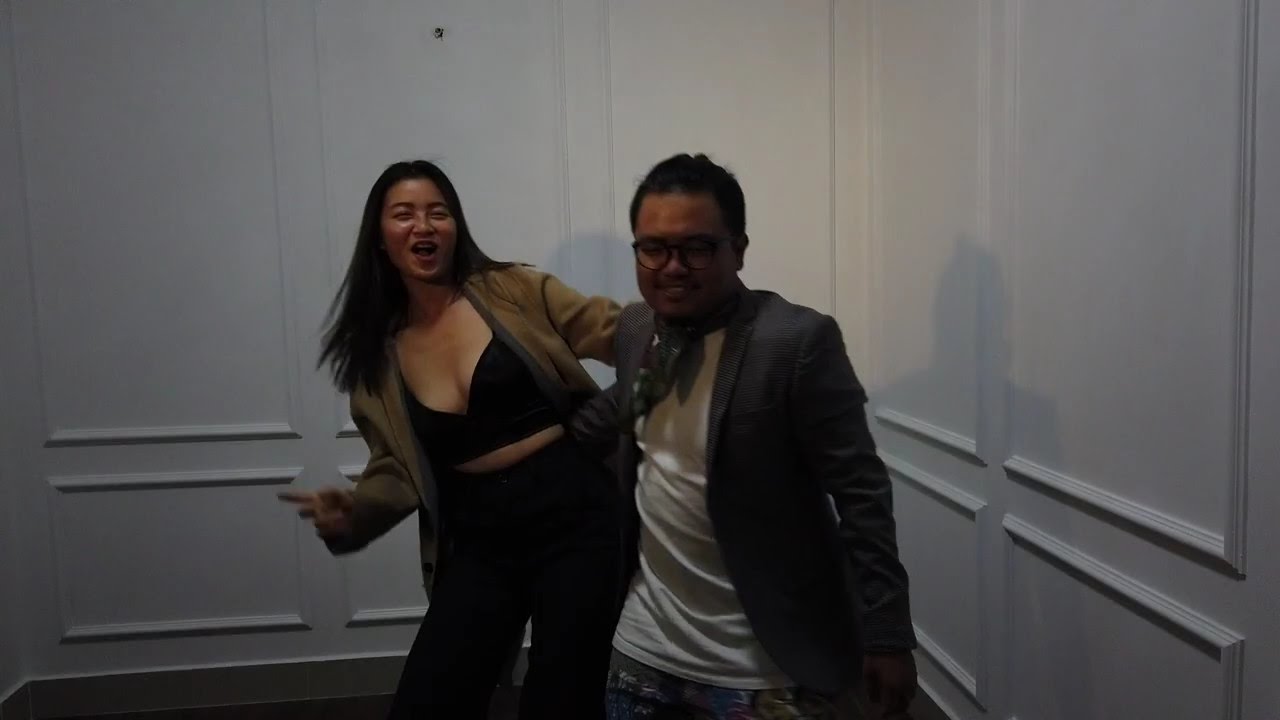This color photograph, taken in landscape orientation, captures a young woman and a young man of Asian descent standing side by side in the center of a small room with white paneled walls. The woman on the left is striking a playful pose, flashing a peace sign with her right hand and smiling or laughing with her mouth open. She has long chest-length dark hair and is dressed in a black crop top or bustier, dark pants, and a tan-colored jacket with black trim. The man on the right, who has short dark hair and wears black-framed glasses, is dressed in a white t-shirt paired with a dark gray suit jacket and torn blue jeans. Adding a stylish flair, he sports a printed scarf tied around his neck. Their interaction appears friendly and casual, with the woman possibly holding a drink or another object in her hand. The room's floor is dark, and a small hole above the woman's head hints at a spot for a painting or decoration. The lighting in the image is somewhat dim, likely enhanced by a camera flash, giving it a slightly dramatic and intimate feel.